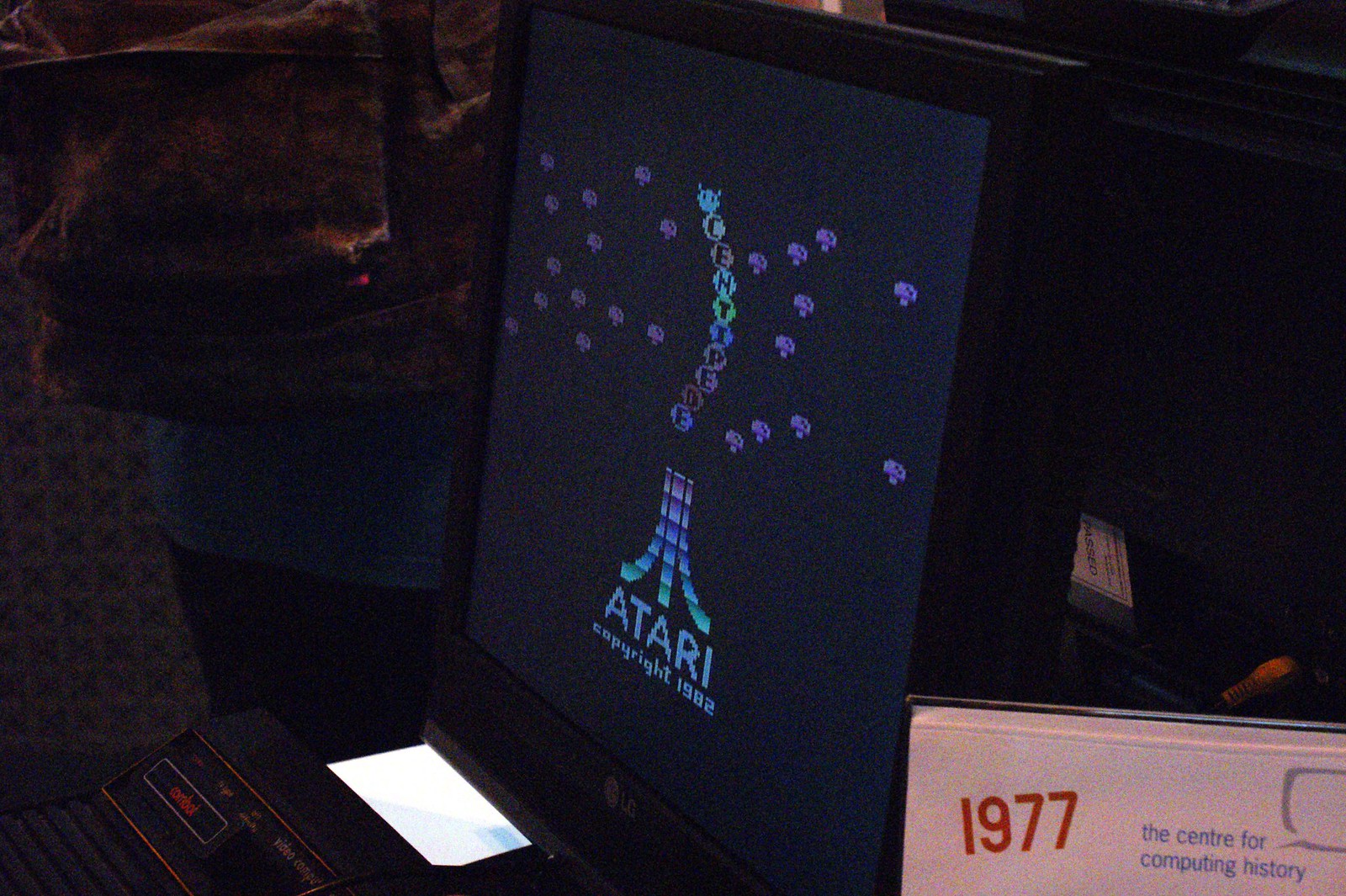In this horizontally-oriented rectangular photograph set against a very dark background, we are presented with a vintage scene. At the center of the image, an old-fashioned Atari screen or packaging prominently displays "Atari © 1982," evoking nostalgic feelings with its retro design. In the lower right corner, the top edge of an open textbook is visible. The textbook features red print in the top left corner that reads "1977," while to the right, blue print on the white paper states "The Center for Computing History." The detailed elements and historical references combine to create a rich tableau that honors the legacy of early computing and gaming.